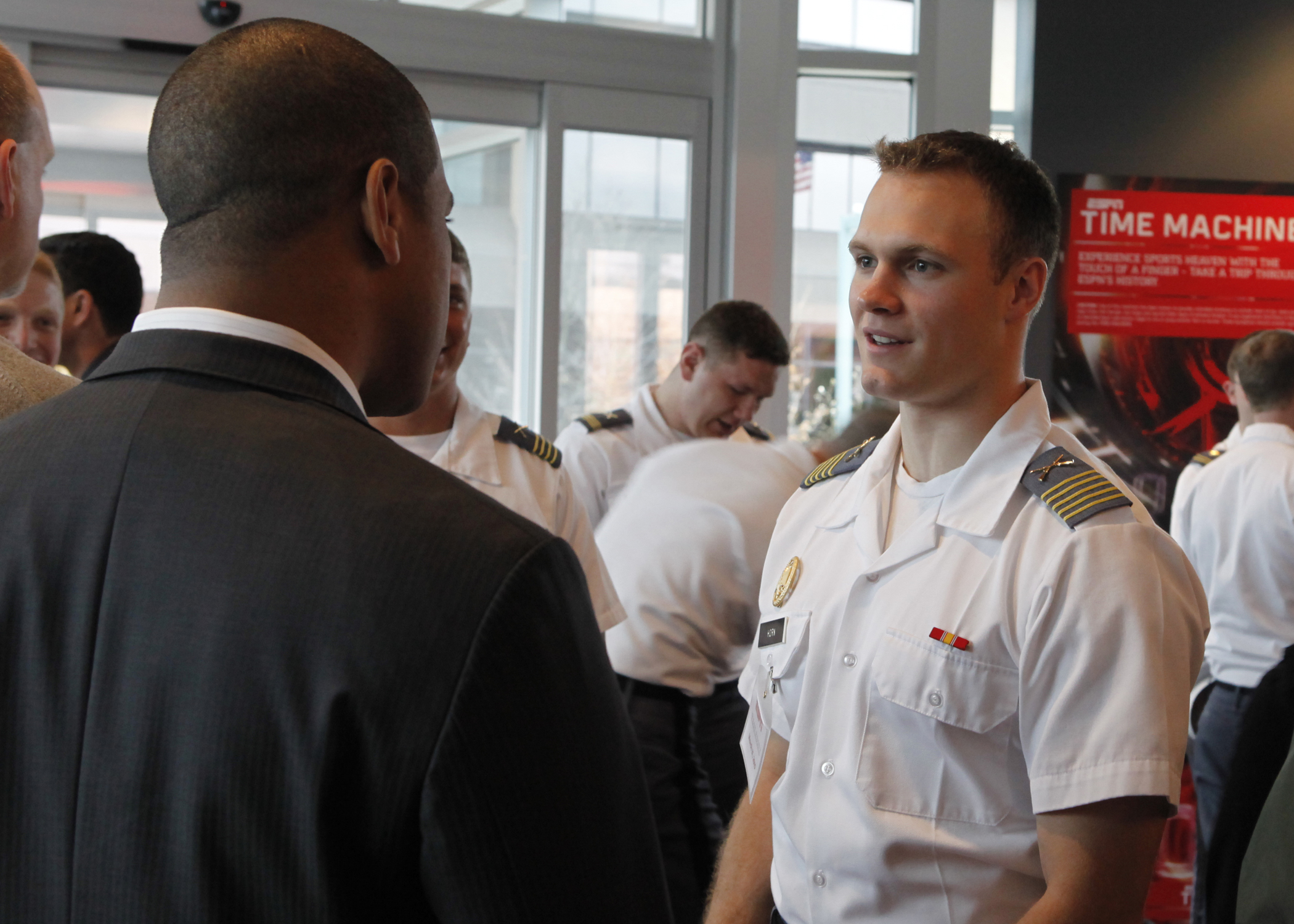The image depicts a bustling scene, possibly in an airport or an indoor establishment, with a cinematic quality to its lighting and texture, suggesting it could be from a film. The central focus is on several men wearing pristine white uniforms, likely military, characterized by white collared shirts with buttoned pockets. They have distinctive patches on their shoulders, adorned with yellow stripes and brass pins featuring crossed symbols. Notably, each individual has a red and yellow stripe above their right shirt pocket, along with a circular badge and a black name tag. 

In the foreground, a young man with short-cropped hair is engaged in conversation with an African American man in a black suit and white collared dress shirt, whose back is turned to the camera. This young man wears the same detailed white uniform as the others, with gold insignia on his chest and a brass pin. The background reveals more individuals in similar uniforms and a partially visible poster mentioning a "time machine," hinting at a thematic element in the setting. Amidst this array of uniformed personnel, the scene conveys an organized yet dynamic atmosphere.